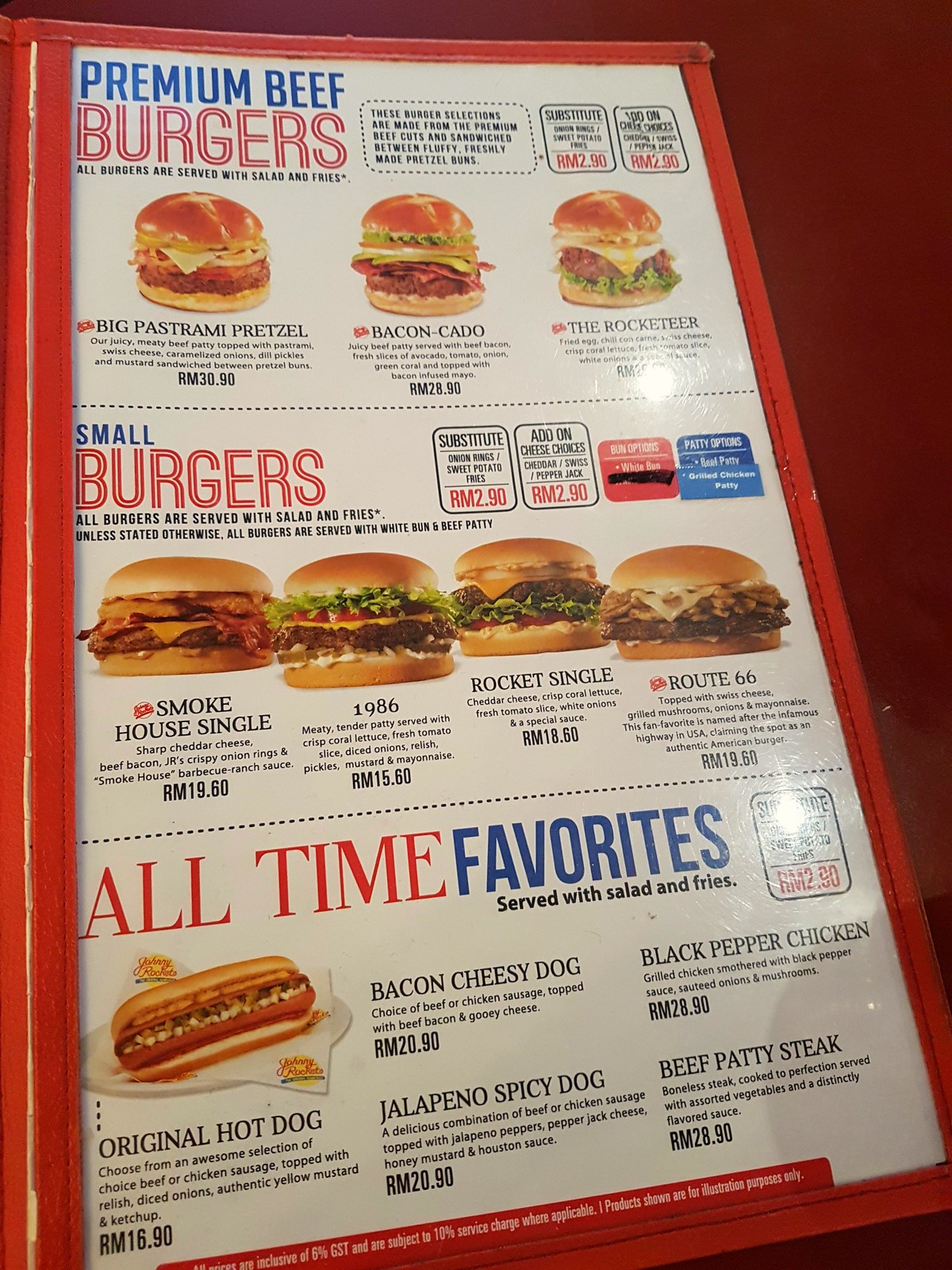This photograph captures a restaurant menu encased in a plastic folder with a red-edged border, giving it a distinct, neatly-organized appearance. The menu features three main sections, each with eye-catching headings and detailed descriptions of various dishes.

At the top, the heading "Premium Beef Burgers" showcases "Premium Beef" in blue and "Burgers" in red font. Below this heading are three enticing burger options, each accompanied by a vibrant image and detailed description:

1. **Big Pastrami Pretzel**: A hearty sandwich featuring a beef patty topped with pastrami, melted cheese, and possibly onions, all encased in a bun. Priced at RM 30.90.
2. **Bacon K-Dough**: A mouth-watering burger with a beef patty, bacon slices, pickles, onion, and lettuce on a bun. Priced at RM 28.90.
3. **Rocketeer**: This burger includes a beef patty and a runny-yolk fried egg dripping down the sides of the bun, though the price is not visible in the image.

A dotted line separates this section from the next, which is titled "Small Burgers". Here, "Small" is in blue font and "Burgers" in red, followed by additional information in black font stating, "All Burgers Are Served With Salad and Fries, Unless Stated Otherwise. All Burgers Are Served With White Buns and Beef Patty." Options for substitutions and add-ons are mentioned but not fully legible. This section highlights four specialty patties:

1. **Smokehouse Single**: Priced at RM 19.60.
2. **1986**: Priced at RM 15.60.
3. **Rocket Single**: Priced at RM 18.60.
4. **Route 66**: Priced at RM 19.60.

The final section, separated by another dotted line, is labeled "All Time Favorites" with "All Time" in red and "Favorites" in blue, and notably mentions that all items are served with salad and fries. This section lists a variety of popular choices, each paired with a picture:

1. **Original Hot Dog**: Priced at RM 16.90.
2. **Bacon Cheesy Dog**: Priced at RM 20.90.
3. **Jalapeno Spicy Dog**: Priced at RM 20.90.
4. **Black Pepper Chicken**: Priced at RM 28.90.
5. **Beef Patty Steak**: Priced at RM 28.90.

The organized layout, color-coded headings, and detailed pictures and descriptions make this menu visually appealing and user-friendly for restaurant patrons.